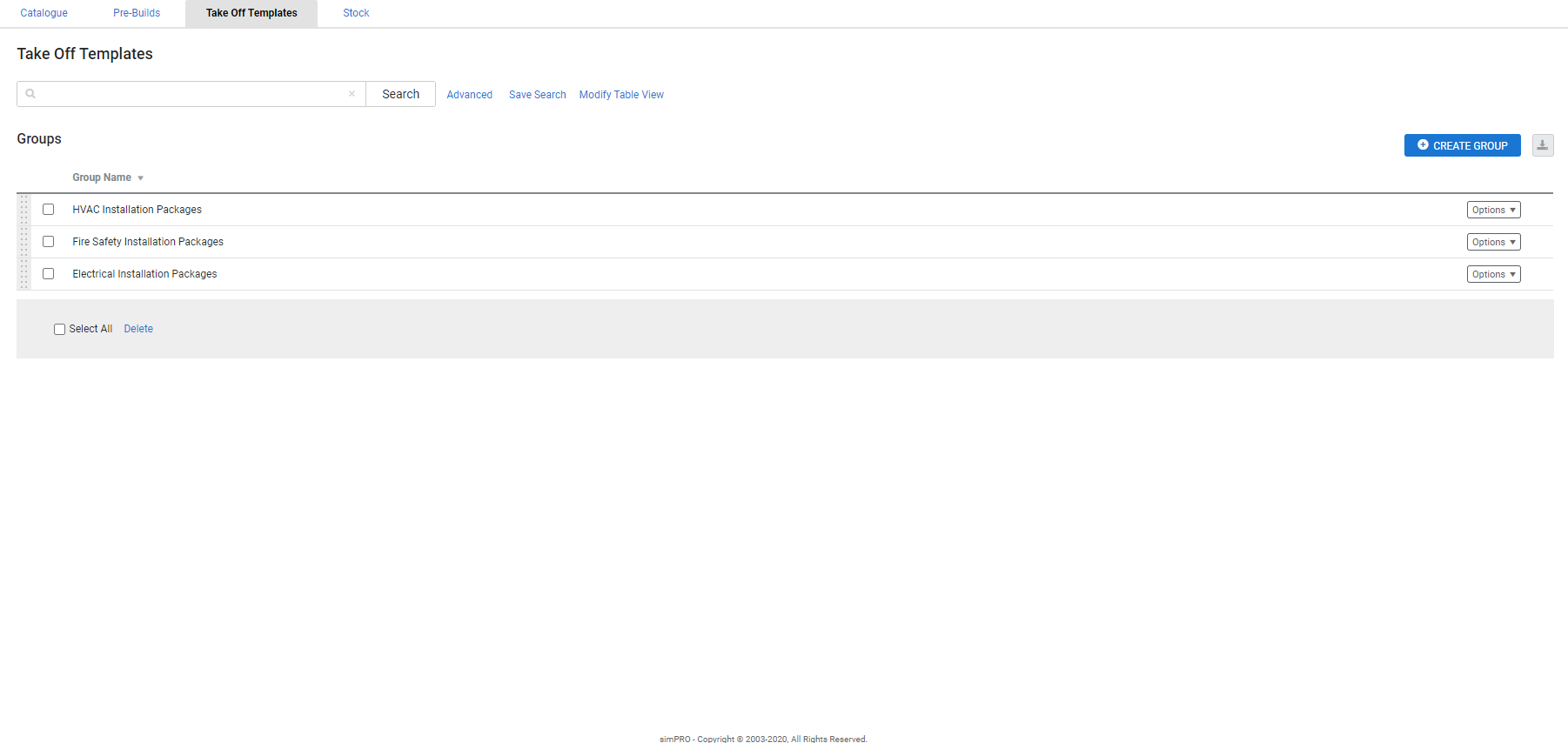The image depicts a detailed interface of the SimPro website, showcasing a catalog at the top, followed by sections labeled "Pre-Builds" and "Takeoff Templates," with the latter being actively selected. A search box is prominently displayed, allowing users to search for specific templates. Below the search box, links for "Advanced Search," "Save Search," and "Modify Table View" are available for user interaction.

The interface is divided into groups, with headers marked "Group Name," listing HVAC Installation Packages, Fire Safety Installation Packages, and Electrical Installation Packages. Each group has an associated set of options accessible via drop-down menus, all labeled "Options," located on the right-hand side.

At the bottom of the interface, there is a gray rectangle housing buttons for "Select All" and "Delete." The "Select All" button is accompanied by a checkable box and is displayed in black, whereas the "Delete" button is highlighted in blue for emphasis. Additionally, a blue "Create Group" button is positioned above the options column.

The bottom-most part of the website features a footer with the text "SimPro Copyright 2003 to 2020 All Rights Reserved," indicating the ownership and copyright details of the site.